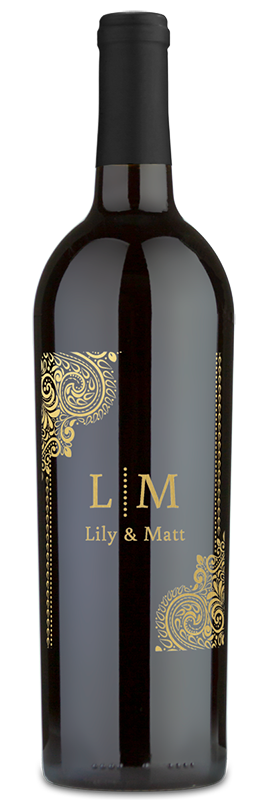This image showcases a sleek black wine bottle set against a stark white background, creating a striking contrast. The bottle, conforming to a standard wine bottle shape, is predominantly black and features an intricate gold design. The gold ornamentation includes a vertical paisley scroll on the top left that extends to the right, mirrored by an identical design on the bottom right that extends to the left. In between these ornate designs are the capital letters "L.M." in gold, followed by "Lily and Matt" written in the same gold serif font. This suggests that the bottle may be a custom piece, such as a wedding souvenir. The bottle remains sealed with an all-black cap, giving it a finished and untouched appearance. The overall look is elegant and festive, making it a sophisticated keepsake.